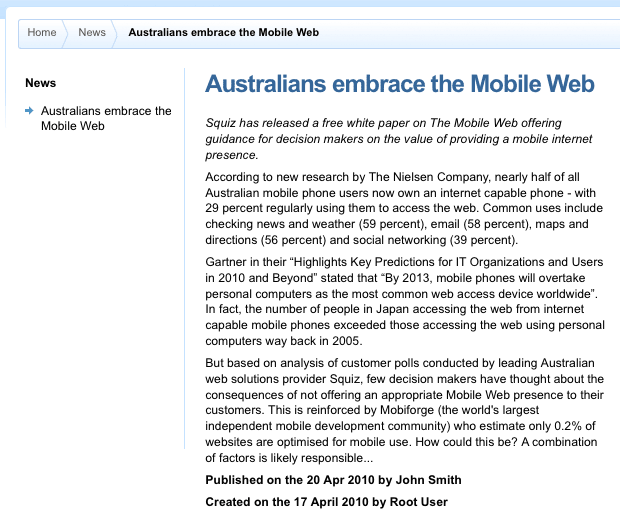This is a detailed and comprehensive caption for the image described:

The image depicts a news webpage with a visually appealing design. The border of the page is sky blue, while the top banner is a lighter shade of blue. Positioned at the top are tabs labeled "Home" and "News." Below these tabs, prominently displayed, is the headline "Australians Embrace the Mobile Web." On the left side of the page, under the headline, there appears another "News" section accompanied by a right-facing blue arrow pointing towards the same headline text, "Australians Embrace the Mobile Web." 

To the right, graced in blue text, is the title "Australians Embrace the Mobile Web," affirming the headline's repeated importance. Below this title lies the body of the article written in standard dark black text. Additional details at the bottom of the article denote that it was published on April 20, 2010, by John Smith and initially created on April 17, 2010, by Root User, further highlighting its credibility and timeliness. This webpage is dedicated to Australian news, showcasing a thorough article on how Australians are increasingly adopting mobile web technologies.